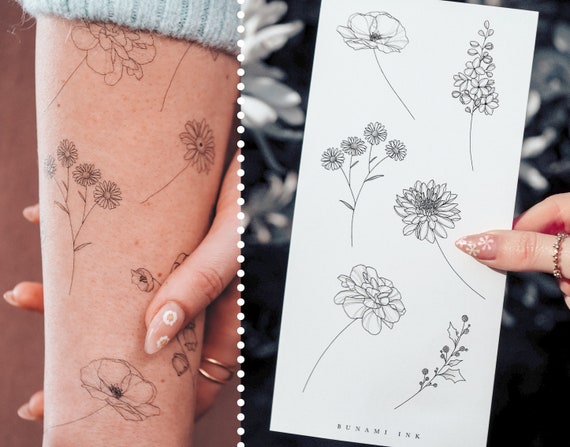The image showcases a woman's left arm adorned with several delicate and dainty floral tattoos, primarily featuring daisies. Her nails, painted pale with intricate flower designs, add to the whimsical theme. She wears gold rings, including a ring on her thumb, adding a touch of elegance to the scene. Part of her blue sweater is visible on her arm. To the right, a white card displays identical floral designs to the tattoos, marked with the text "Tsunami Inc." This suggests that the tattoos are likely decals from this brand, seamlessly transferred onto her arm. These temporary tattoos, which can be washed off in due time, offer a beautiful and subtle adornment without the permanence of traditional tattoos.